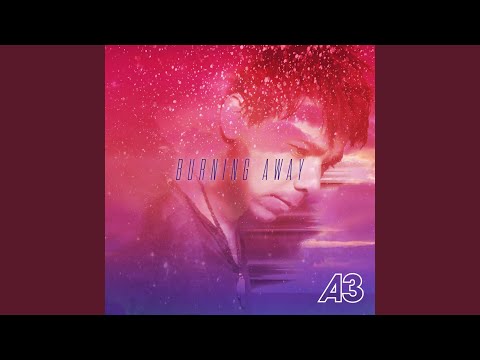The image is a graphic likely intended as a cover for a CD or album. It is oriented in a landscape manner with black banners on the top and bottom, and vertical maroon banners on the left and right. In the center, a colorful gradient transitions from a reddish pink at the top, through shades of pink and purple, to a darker purple at the bottom. Within this gradient, there is an image of a man shown from the biceps up, with short dark hair, looking downwards and to the right, his expression somber. Overlaying the image, in italicized capital letters and a purple font, is the text "BURNING AWAY." In the lower right corner, the text "A3" appears in white, set against the colorful background. Overall, the composition suggests it could be a front cover for an album or EP.